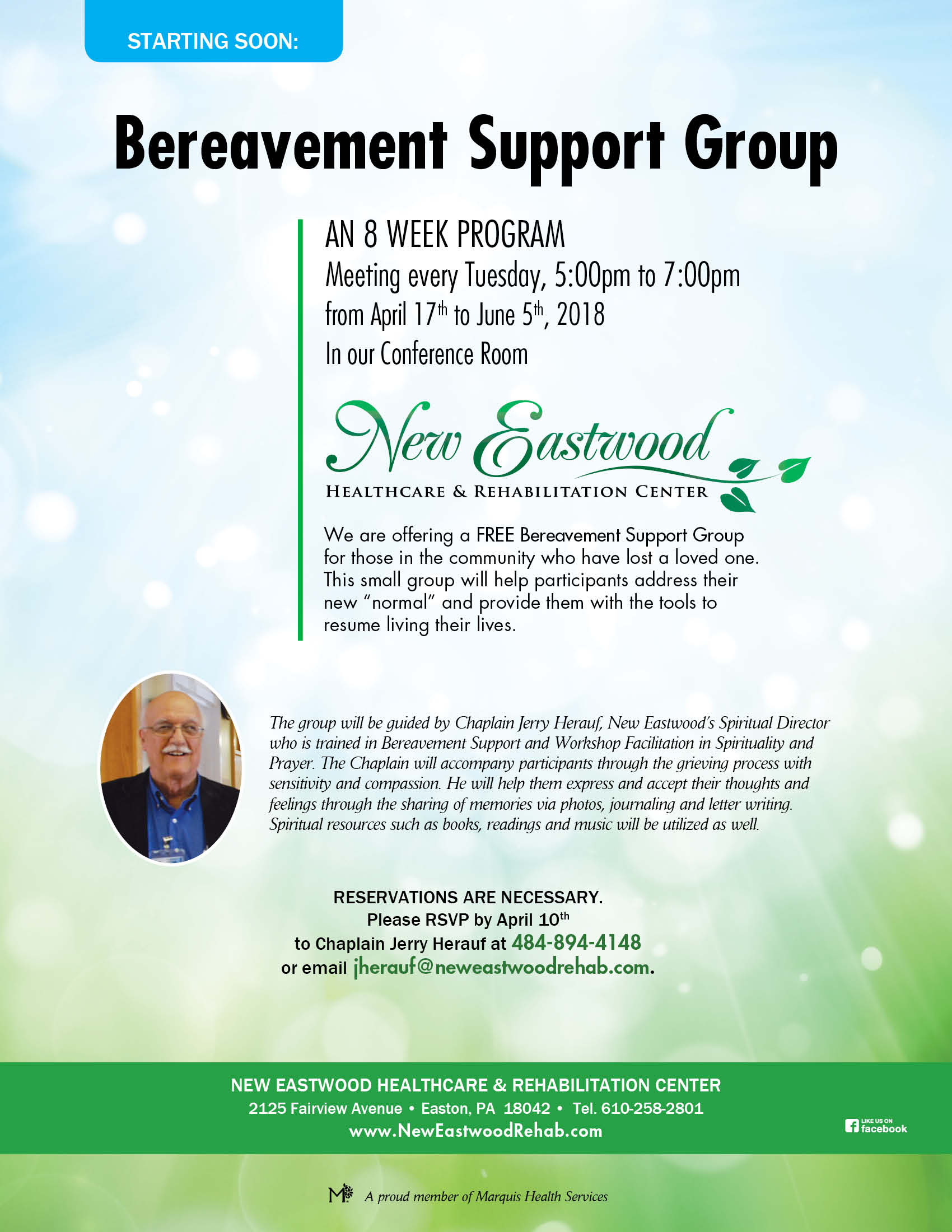This image is a detailed pamphlet for a bereavement support group set against a backdrop that transitions from a blue sky at the top to green at the bottom. At the very top, the phrase "Starting Soon" is prominently displayed in white lettering within a blue box. Below this, the title "Bereavement Support Group" stands out in bold black text. The pamphlet details an eight-week program meeting every Tuesday from 5 p.m. to 7 p.m., starting April 17th and ending June 5th, 2018, taking place in the conference room of New Eastwood Health Care and Rehabilitation Center.

A green vertical line flows down the side, and beside it, in green cursive-like lettering, the words "New Eastwood" are featured, followed by "Health Care and Rehabilitation Center" in black text. An illustration of a green swoosh with green leaves appears next to this text.

The pamphlet elaborates on the offer of a free bereavement support group for community members who have lost a loved one. The support group aims to help participants address their new normal and provide tools to help them resume their lives. The group is overseen by Chaplain Jerry Holliff, New Eastwood's Spiritual Director, who is trained in Bereavement Support and Worship Facilitation. He will guide participants through the grieving process with sensitivity and compassion, helping them express their thoughts and feelings through various activities such as sharing memories via photos, journaling, and letter writing. The use of spiritual resources like books, readings, and music will also be incorporated.

An elderly man with white hair, a white mustache, a blue shirt, and a black jacket is featured in the bottom corner of the pamphlet. At the very bottom, a green bar contains all the contact information: New Eastwood Health Care and Rehabilitation Center, 2125 Fairview Avenue, Easton, PA, 18042, telephone 610-258-2801, and the website www.neweastwoodrehab.com. Reservations are required, and those interested are asked to RSVP by April 10th to Chaplain Jerry Holliff at 484-894-4148 or via email at jerryholliff@neweastwoodrehab.com.